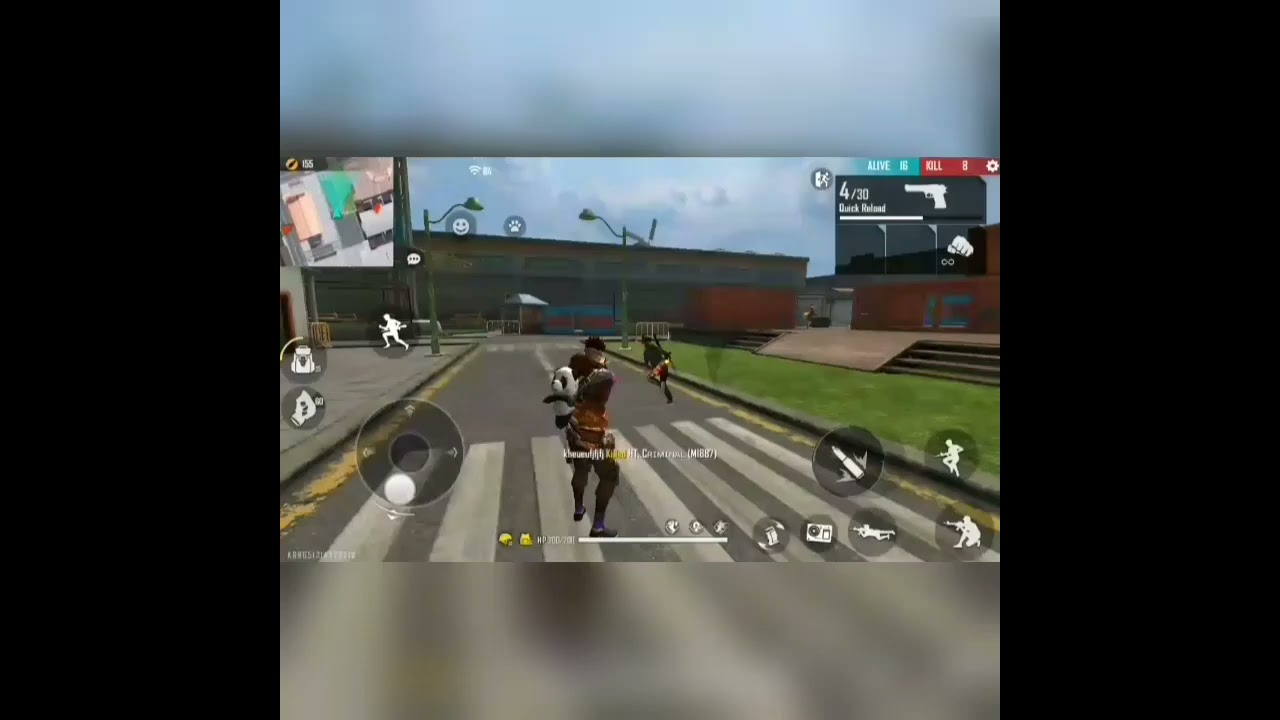This is a screenshot of a video game, resembling Fortnite, featuring an urban street scene with various buildings, grassy patches, and street lamps. A main character stands directly in front, centered in a crosswalk, wearing tight pants, a shirt, a military-style belt, and a helmet, holding a plush panda. To the right of this character, another figure is running. The scene includes several black and white action buttons on the screen's bottom-right, depicting a kneeling shooter, a jumping shooter, a running character, a rocket, and a laying down shooter. There's also a joystick-like control knob on the left, along with multiple icons, such as a camera and bullets. A help bar is visible at the bottom, and an ammo counter displaying "430" is positioned at the top right. The interface shows a mix of additional game information, like a map on the top left and various utility icons. The background features a sunny sky above buildings and a significant grassy area, contributing to the outdoor setting of the game.